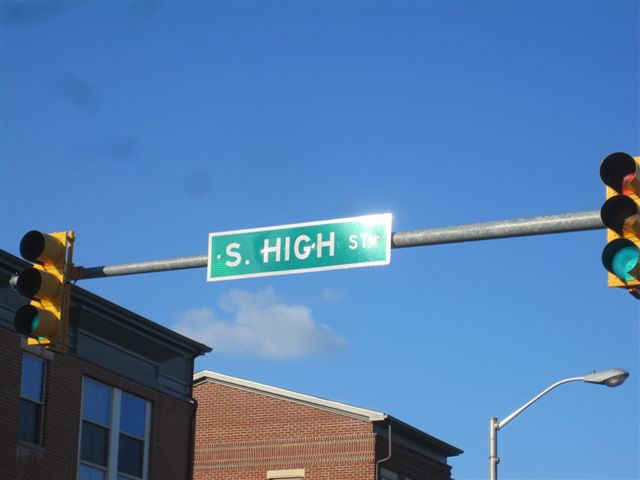This image captures a traffic signal mounted on a pole that extends over the lane of oncoming traffic. The traffic signal at each end of the pole displays a green light, while the red and yellow lights above them remain unlit. Between these traffic signals is a green street sign with a white border that reads "S. High Street." In the background, a solitary street light and two brick buildings with white windows and trim are visible. The scene is set against a backdrop of a beautiful, clear blue sky adorned with a single small, puffy white cloud.